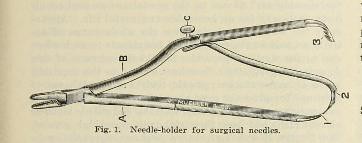Figure 1: Needle Holder for Surgical Needles

This black and white illustration, appearing on yellowish paper indicative of an older book or textbook, depicts a detailed sketch of a surgical tool known as a needle holder. The artwork, seemingly crafted with pencils, captures the intricate design of the instrument used in surgical procedures. Various parts of the needle holder are labeled with alphanumeric markers including letters (A, B, C) and numbers (1, 2, 3); however, the corresponding explanations for these labels are not included in the image. This meticulous representation highlights the precision and importance of the tool in medical contexts.